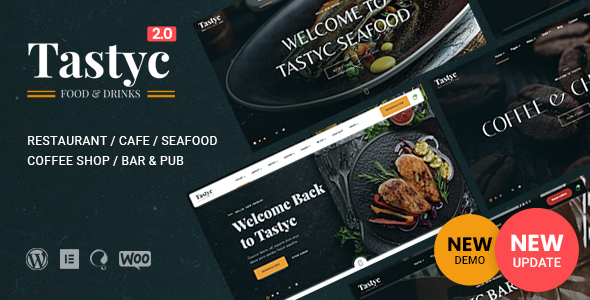**Caption:**

Welcome to Tasty C Seafood Restaurant! In the top right corner of the image, there is a red circle displaying the words "2.0," indicating a new update. The backdrop of the image is predominantly black, complementing the restaurant's modern color theme. 

In the bottom left, the text "WordPress" is visible next to a set of headphones. The header of the image warmly welcomes diners back to Tasty C, showcasing a variety of dishes including succulent meat, fresh veggies, and artful plating that highlights the restaurant's seafood specialties. Alongside the food, there's a glimpse of coffee and other beverages, hinting at the establishment's diverse offerings as a restaurant/cafe/seafood venue, and also functioning as a coffee shop, bar, and pub.

Bright, vibrant colors dominate the visual, with peppers and assorted vegetables adding a pop of freshness. The orange circle with black text announces a "new demo," emphasizing Tasty C's ongoing innovations.